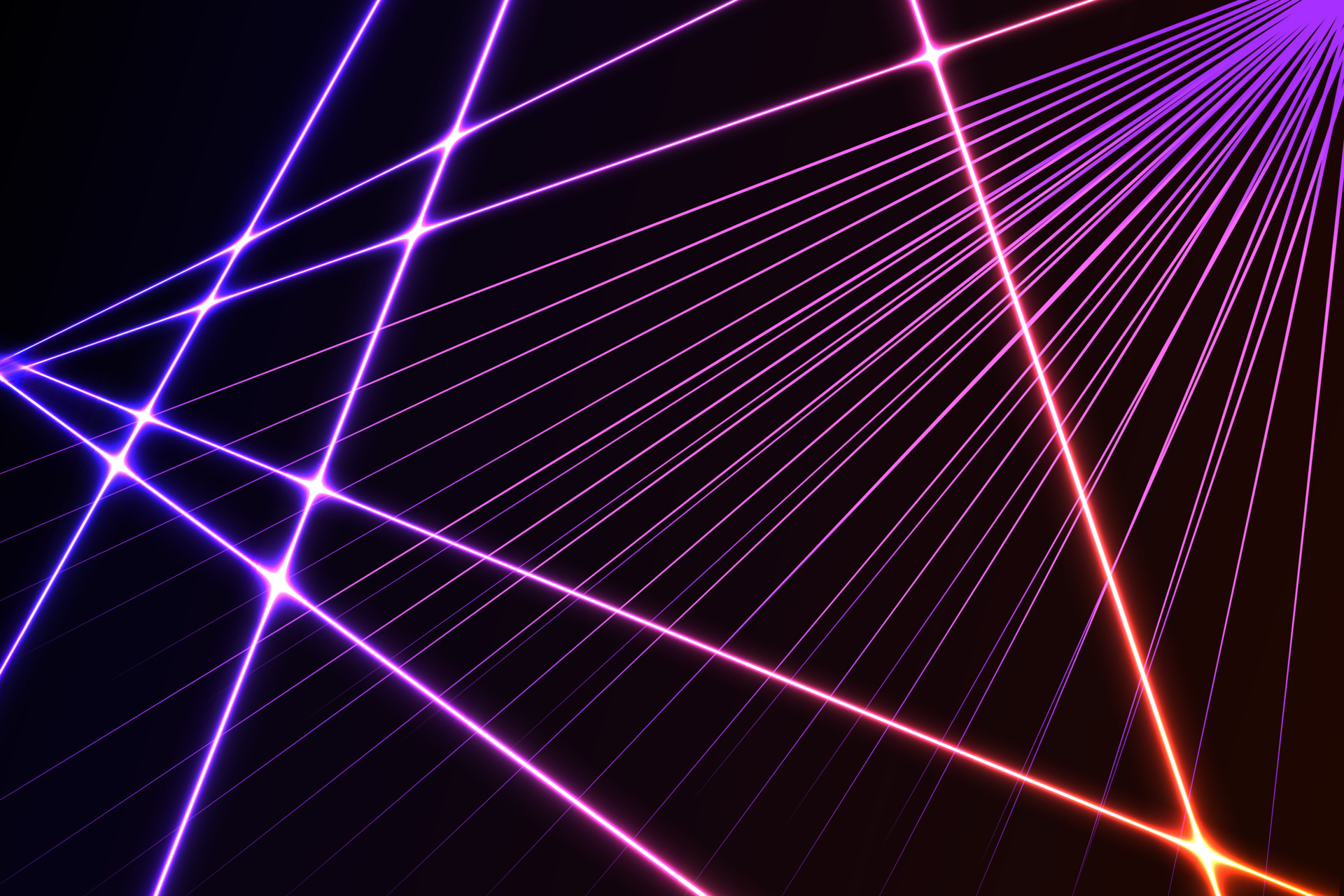The image captures a vibrant digital illustration reminiscent of a laser light show, set against a black background. Numerous laser beams, primarily in shades of purple, mauve, lavender, and red, radiate from the top right corner, spreading diagonally across the image towards the bottom left. These beams vary in width and intensity, with some fading into pink hues before eventually returning to purple and black as they descend. Among them, thicker parallel lines begin on the left side and extend horizontally and diagonally in neon orange and purple shades. The composition also features vertical and horizontal intersections, highlighted by bright white points where they intersect. Notably, three triangular laser beams in shades of reddish, mauve, and blue descend from the top, while a singular red beam emerges from the bottom right, crossing multiple lines as it ascends towards the left. Additionally, four purple-red beams originate from the middle left, extending upwards and downwards at sharp angles, contributing to the striking visual complexity of the scene.